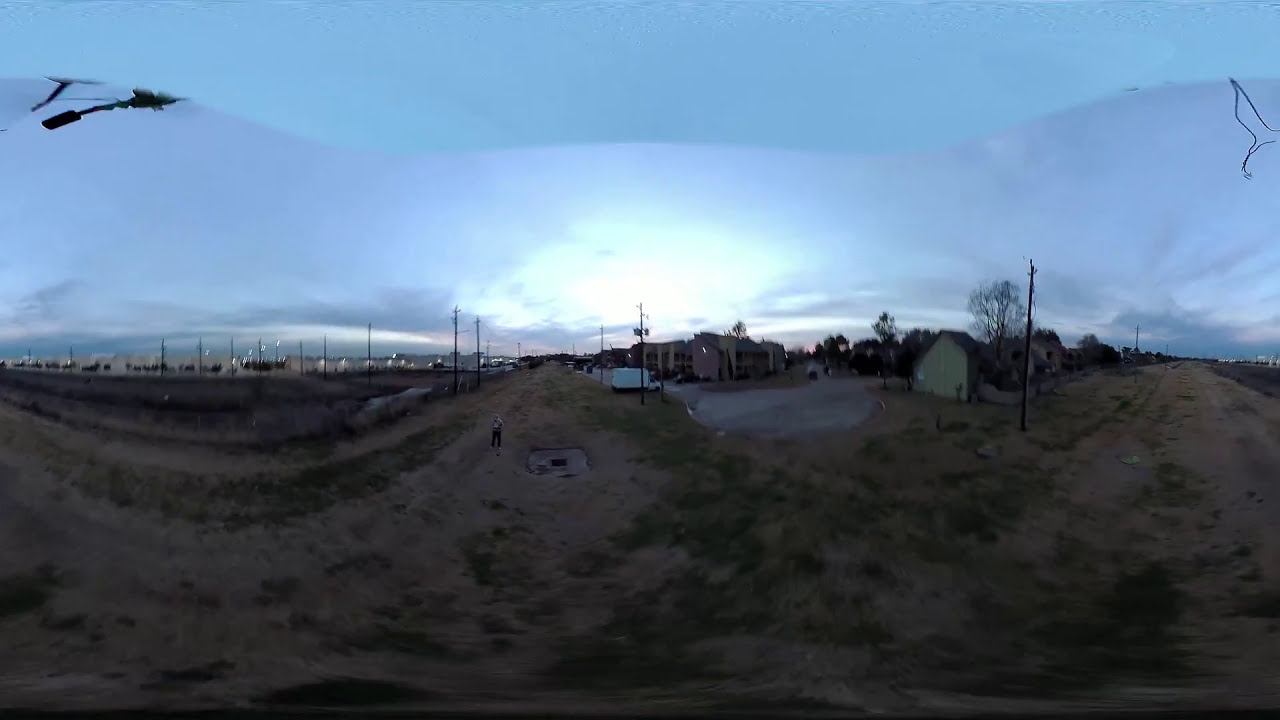The image appears to be a digitally altered or drone-captured 360-degree panoramic view of a rural area, showing a town with a variety of buildings, including an industrial complex far in the background. The image is characterized by its vivid and somewhat distorted details, with a bright sky in the center transitioning to a bluish-teal hue towards the edges. A notable line cutting across the sky suggests possible post-editing. In the foreground, the scene reveals a dirt road that curves to the right, leading towards an indistinct destination, with hilly, barren terrain dominating the front. Power lines crisscross the sky above, and to the right, there's what looks like a garage or farmhouse. Despite its rural setting, traces of suburban development, such as apartments, are visible, adding to the site's varied landscape. The time of capture seems to be either early morning or late evening, inferred from the low position of the sun. The overall atmosphere is both intriguing and mysterious, drawing attention to the unnatural cutoff in the sky, possibly indicating a technical anomaly or artistic manipulation.